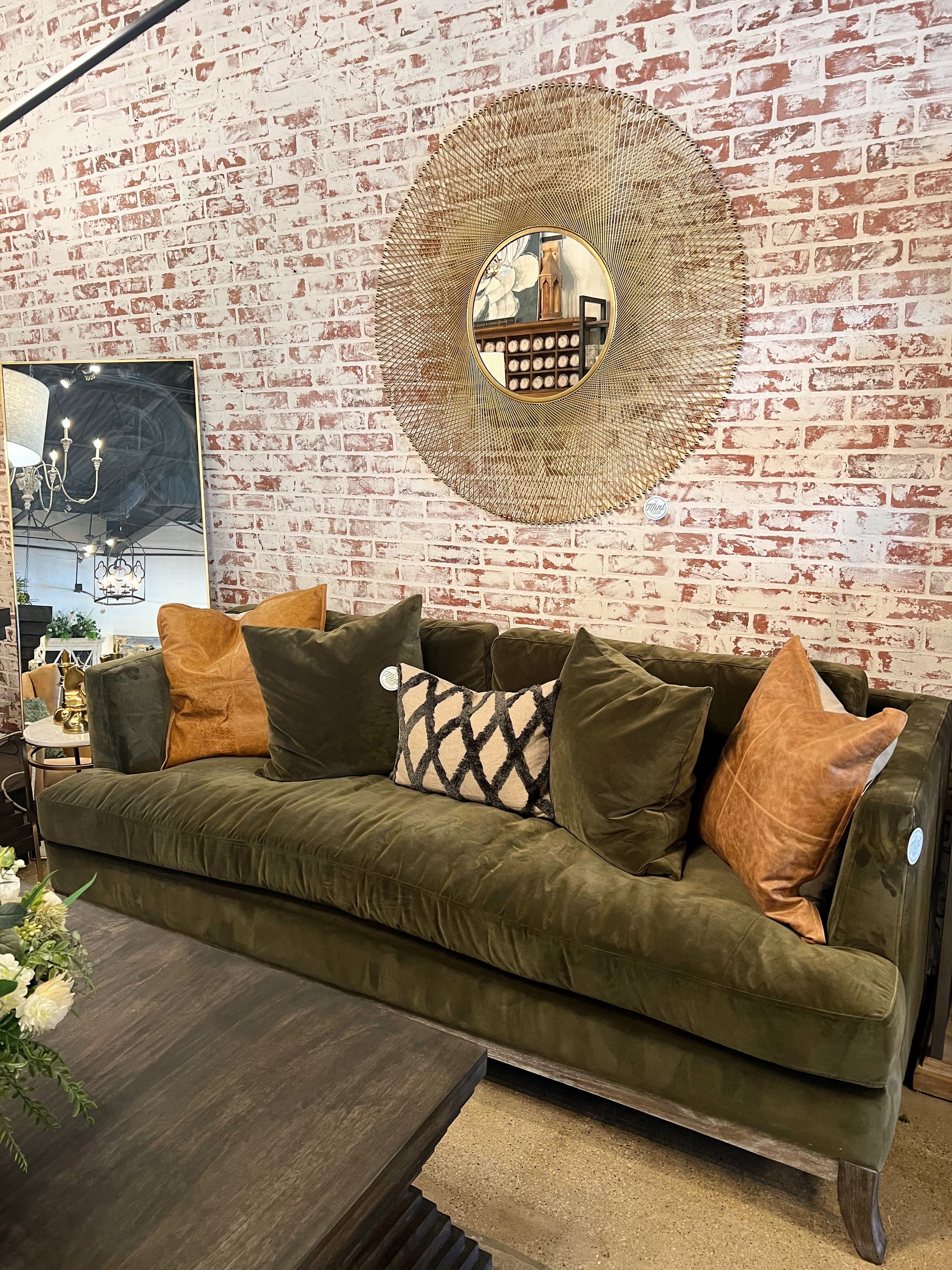This image depicts a meticulously arranged showroom that resembles a cozy living room environment. Dominating the center of the scene, a plush, dark green suede sofa is adorned with numerous cushiony pillows, including a notable beige one and another matching dark green pillow. It intriguingly bears what appears to be a price tag on its right side, reinforcing the impression that this might be a furniture store or an antique shop.

The sofa is set against an exposed brick wall, featuring a mix of chalky white paint offset by patches of traditional red brick, creating a weathered, yet aesthetically pleasing backdrop. To the left of the couch stands a substantial floor mirror, which reflects the expansive showroom, hinting at a warehouse-like space with black roofing visible in the reflection.

Adding to the antique ambiance, a dark brown wooden table is positioned in the bottom left-hand corner of the image. The table, with an antique appearance, partially reveals a plant with green leaves and delicate white flowers, enhancing the room's natural and inviting aesthetic. The showroom is further ornamented with an eye-catching large round mirror on the wall, which features a distinctive fanned-out dial design around it, contributing to the overall vintage charm of the setting.